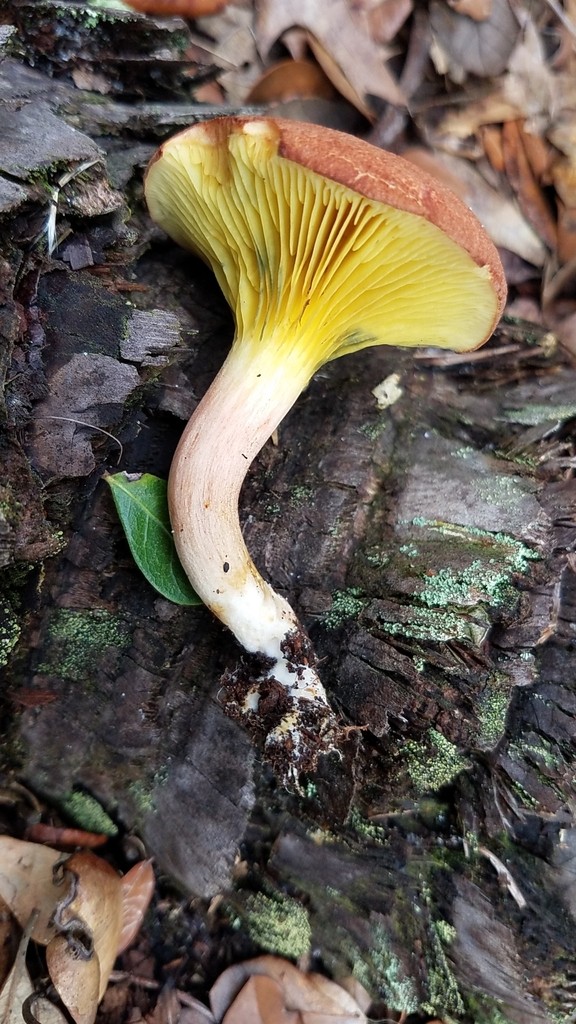The photograph captures a detailed outdoor scene featuring a solitary mushroom centrally positioned on a decayed, horizontally placed tree trunk. The tree trunk, which is dark grey to almost black in color and adorned with patches of green moss, spans diagonally across the image from the upper left to the lower right. The forest floor around the trunk is scattered with brown, dried leaves, contributing to the earthy ambiance.

The mushroom has a curved whitish-beige stalk that emerges from the decaying log. The stalk, about an inch and a half in height and half an inch in width, inclines to the left before curving back to the right. The cap of the mushroom, which is a distinct reddish-brown, partially reveals its yellow gills with thin elongated strands underneath. The mushroom appears deeply rooted in the rotting wood, surrounded by a grey, soil-like substance. A green leaf lies adjacent to the mushroom, contrasting with the browned leaves that litter the background, enhancing the composition's natural and organic feel.